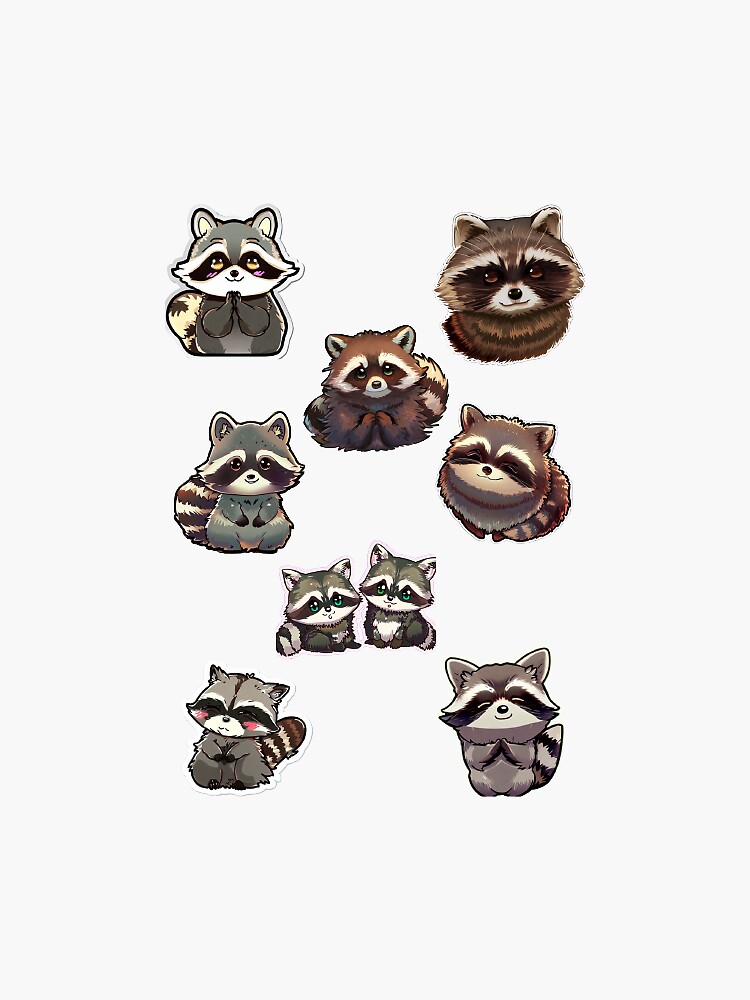The image features a clustered array of nine cartoonish raccoons set against an off-white to light gray background, arranged in what appears to be three columns. These raccoons vary slightly in size and color, predominantly illustrating shades of gray, white, and brown. The raccoons are depicted in various charming and cutesy poses, each showing distinctive characteristics and expressions. 

In the left column, the top-left raccoon has its hands clasped together in a manner resembling prayer and is gazing directly at the viewer. The raccoon at the bottom-left also has its hands together and its eyes closed, giving a gentle, blushing appearance. Their big bushy tails, marked with brown and white stripes, are visible behind them. 

In the middle column, the top raccoon stands out with detailed brown and white fur, again, looking at the viewer with big eyes. Below it, nestled in the center, are the smallest raccoons of the group, distinguished by their larger green eyes and cutesy expressions, each about half the size of the others.

The right column features a raccoon that appears more realistic and furry, positioned at the top with prominent detail. Below this one, another furry raccoon appears with eyes contentedly closed. At the bottom-right, a raccoon mimics the hand-together pose similar to the one in the bottom-left, with closed eyes, and has a more simplistic design.

The entire arrangement creates a visually appealing, artistically-rendered scene of endearing raccoons, each displaying various engaging expressions and poses from clasped hands to intricate fur detailing.